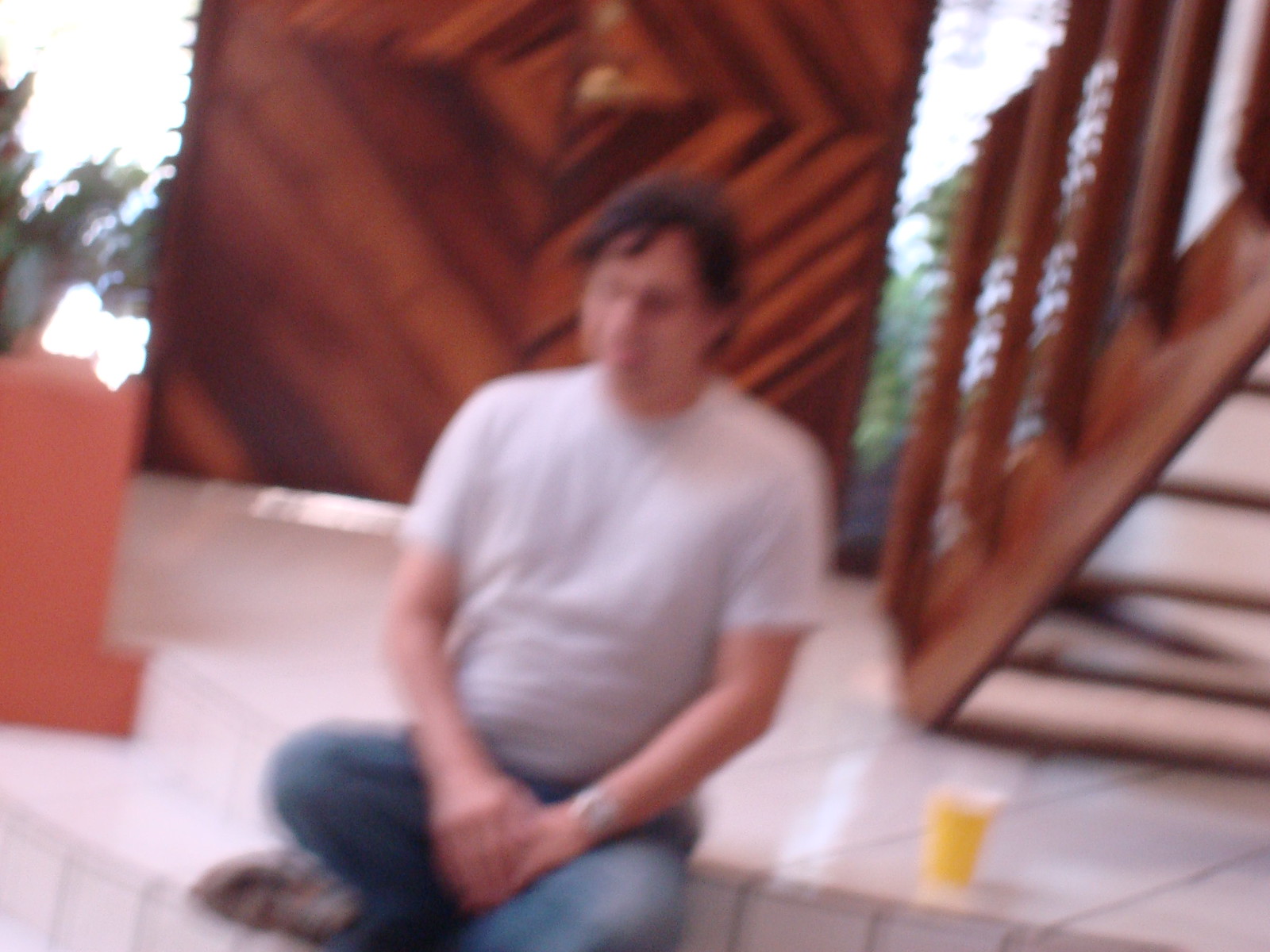In this blurred photograph, a man is seated on a set of interior stairs. The scene appears to be indoors as more wooden stairs ascend behind him to the right, leading to a higher platform. The man, dressed in a gray shirt and blue jeans, sits cross-legged with a cup—possibly containing orange juice—positioned on the tiled floor beside him. The entire image lacks sharpness, obscuring fine details. To his left, large wooden doors with a diamond pattern comprised of various wood hues are visible, suggesting a complex and intricate design.